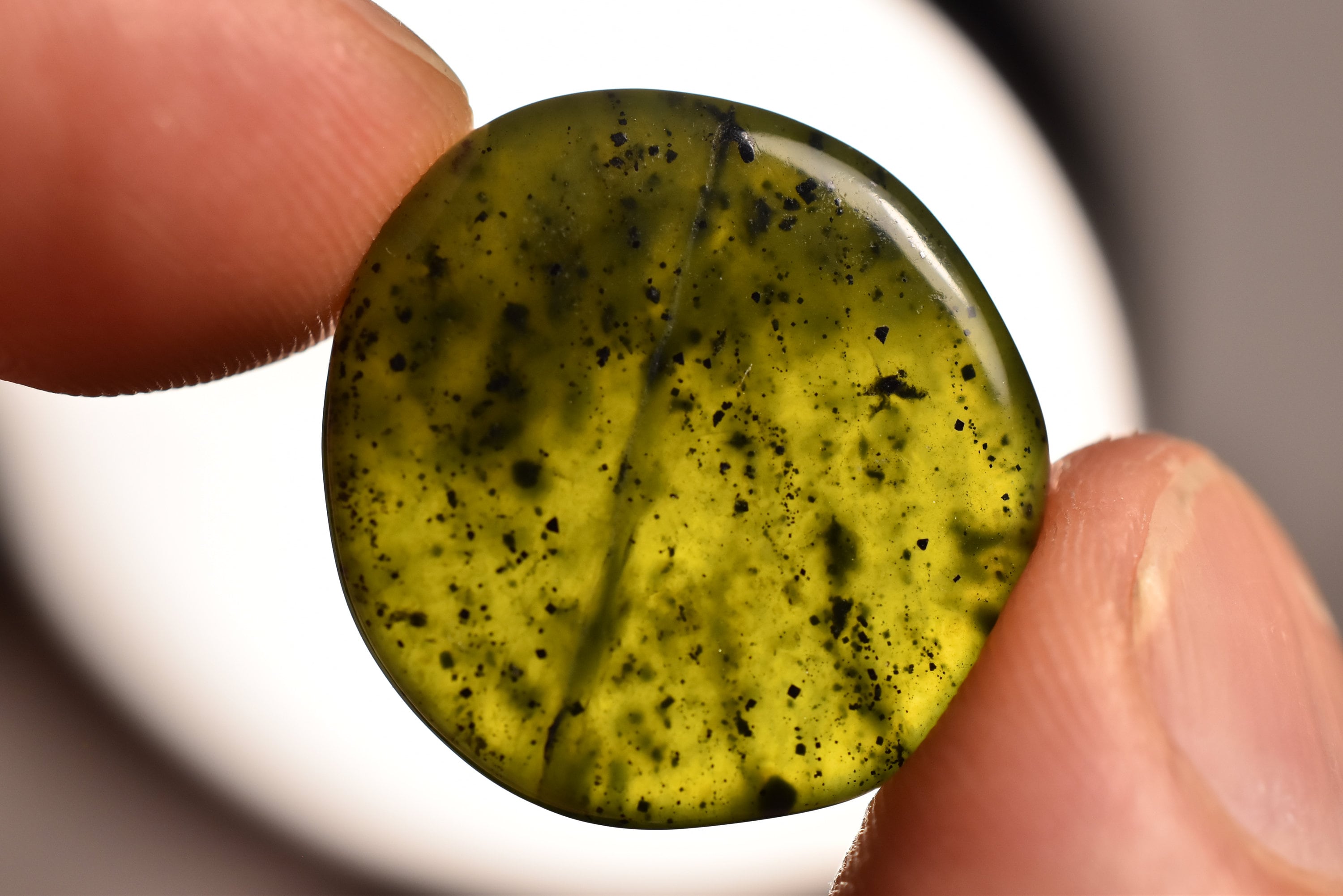This photograph is an extreme close-up of two thumbs holding a small, shiny, translucent disk, likely made of glass. The disk primarily exhibits a yellow hue with numerous black dots and splotches scattered across its surface. Highlights on the disk indicate it is catching light from an external source. The background is out-of-focus, featuring a large white circle, possibly a plate or light, set against a gray backdrop. The thumbs appear to belong to a person with light, pale skin and short-trimmed fingernails, one thumb located in the lower right corner and the other in the upper left corner. This close-up shot accentuates the intricate details of the hands, including fingerprints and nail texture.